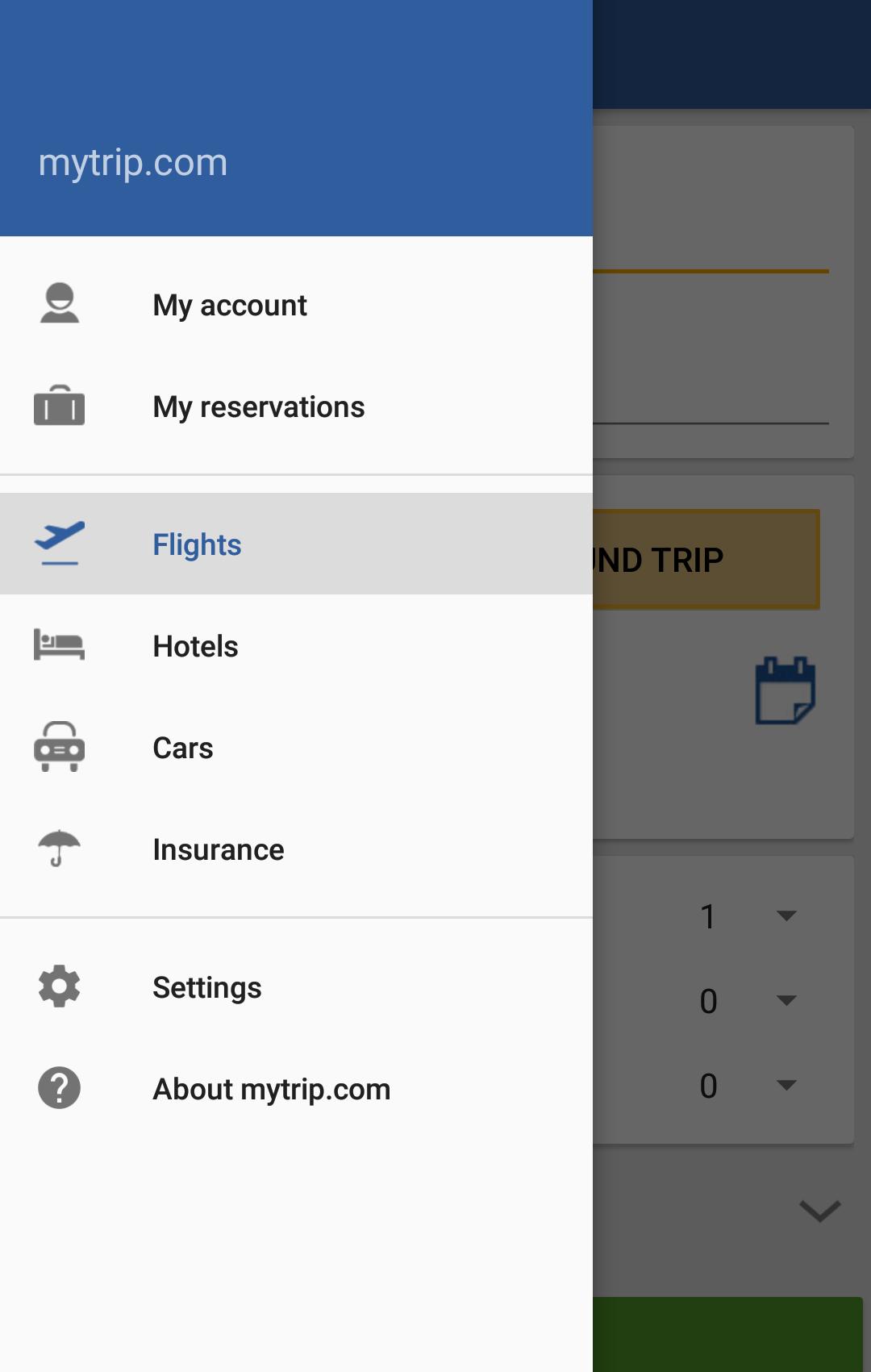The image depicts a vertically-oriented rectangular interface, partially obscured by a gray overlay. In the background, there's a blurred website visible on the right side. On the left side, an expanded menu is present. The menu begins with a blue strip at the top, displaying "mytrip.com" in white text. Below this header, the background is white with a left-justified list of clickable options: "My Account," "My Reservations," "Flights" (highlighted in blue, suggesting current selection), "Hotels," "Cars," "Insurance," "Settings," and "About MyTrip.com." Under the "Flights" option, a thin gray strip is visible, further indicating it is the active section.

Below this, additional elements are partially visible through the overlay. These include several blue lines and a yellow line. A truncated button appears to say "ND trip," though not fully discernible. A blue calendar icon and a series of numbers ("1," "0," and "0") with pull-down menus, presumably in black text, are located on the right side. Under these, there's a larger pull-down arrow in black. The bottom of the interface features a green strip, although its content is indiscernible due to the gray overlay. The overall scene suggests the menu is related to booking or managing flight reservations on a travel website.